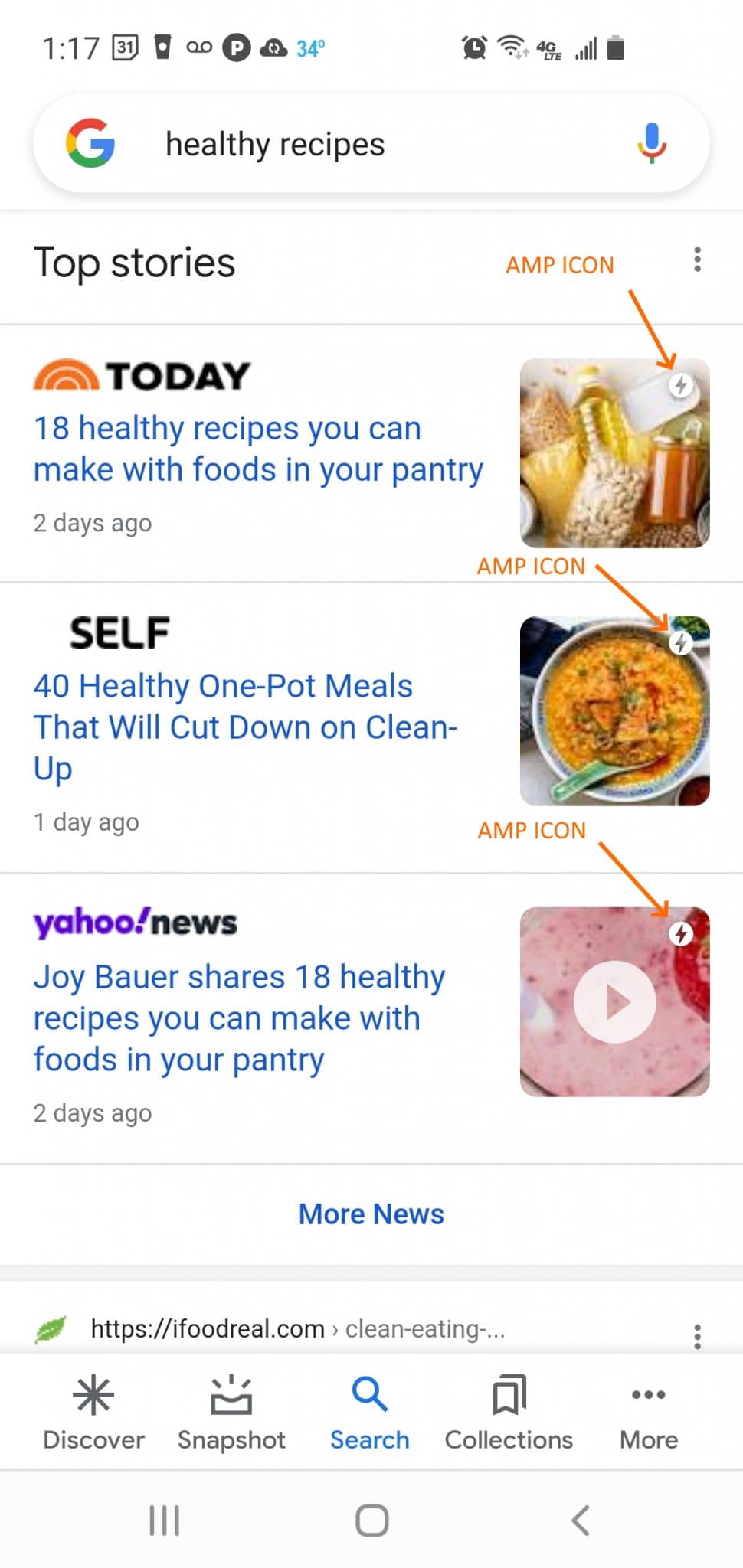A detailed screenshot of a Google search on a smartphone at 1:17 PM, showing a temperature of 34 degrees (unit unspecified). The phone has decent reception and an alarm set. The search query is for "healthy recipes," indicated by the active microphone icon. 

Top stories include:
1. An AMP icon source (likely USA Today) featuring "18 Healthy Recipes You Can Make with Foods in Your Pantry" – emphasizing on preparation with pantry ingredients.
2. Self magazine's article on "40 Healthy One-Pot Meals That Will Cut Down on Cleanup," illustrated with a bowl of soup – ideal for minimizing dishwashing duties.
3. Yahoo News highlights "Joy Bauer Shares 18 Healthy Recipes You Can Make with Pantry Foods," dated two days ago, fitting the theme of easy, pantry-based cooking.

The search page also features options to view more news, visit foodreal.com, and access snapshots, collections, and additional resources.